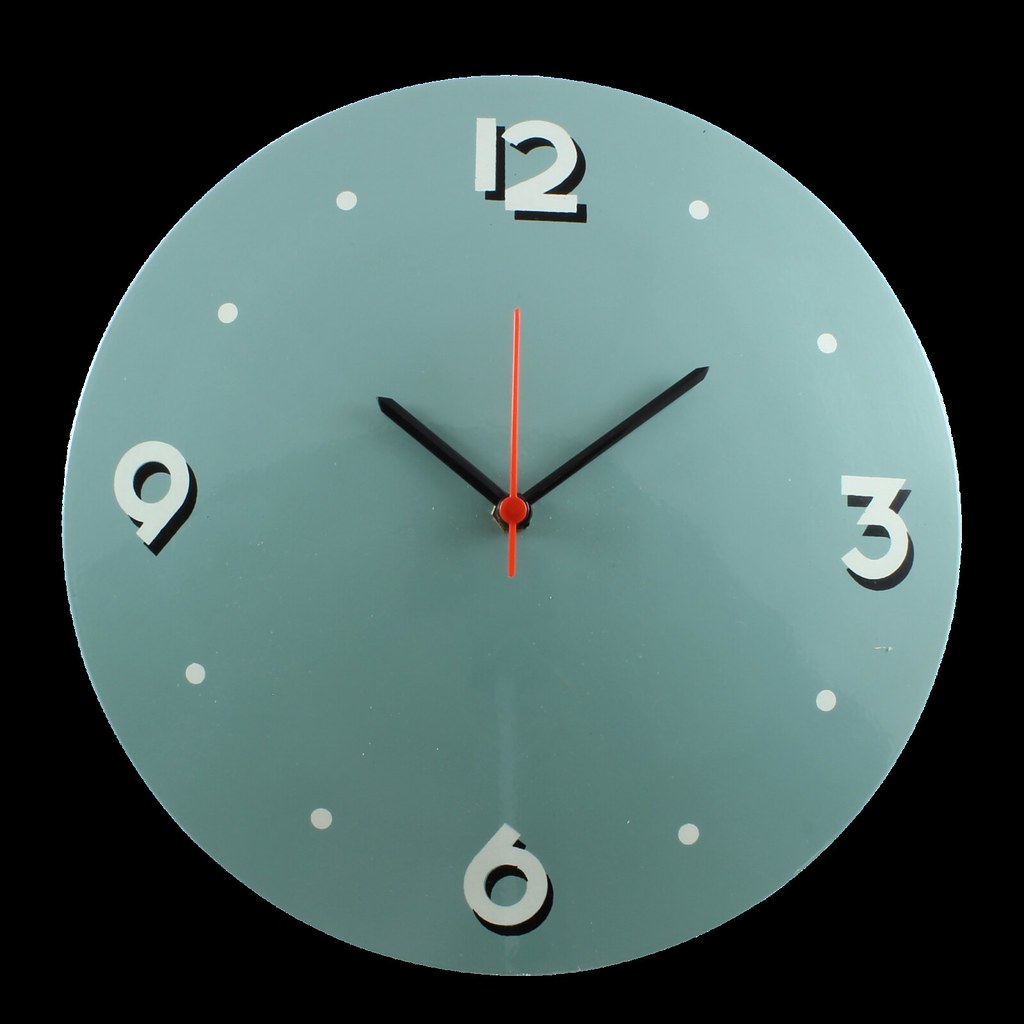The image depicts the face of a vintage-style clock, primarily in a muted teal hue. It lacks an exterior frame, showcasing only the clock's circular face. The numbers 12, 3, 6, and 9 are prominently displayed in a bold, 60s or 70s-style font with significant black drop shadows, while the remaining hours are marked by small dots in a very light teal, almost white color. The hour and minute hands are black, contrasting sharply with the background, and the second hand is red, adding a pop of color. The clock face appears to have been digitally cut out, with its edges displaying pixelation, and is set against a solid black background.